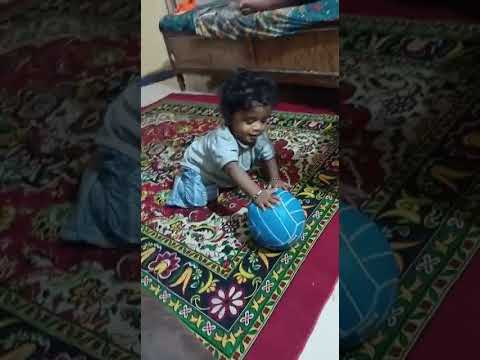This photograph captures an enchanting moment of a young girl, possibly of Indian descent, engrossed in play with a blue and white volleyball on a vividly detailed Persian-style rug. The toddler, who appears to be around one year old, has dark black, curly hair tied into a small ponytail. She is dressed in a gray shirt and blue pants. The intricately designed rug beneath her features a green border adorned with delicate floral patterns in shades of yellow, purple, and white, with the interior marked by a mix of white and burgundy accents forming exquisite floral designs.

The setting appears to be a living room, highlighted by a couch in the background and possibly a bed frame with a comforter visible. The photograph is artistically centered on the girl, with black-tinted, zoomed-in sections of the same image appearing on the left and right sides, adding a dramatic focus and symmetrical balance to the composition. The child's intense concentration on the volleyball as she pushes it along the multicolored rug creates a heartwarming and vivid portrayal of simple childhood joys.